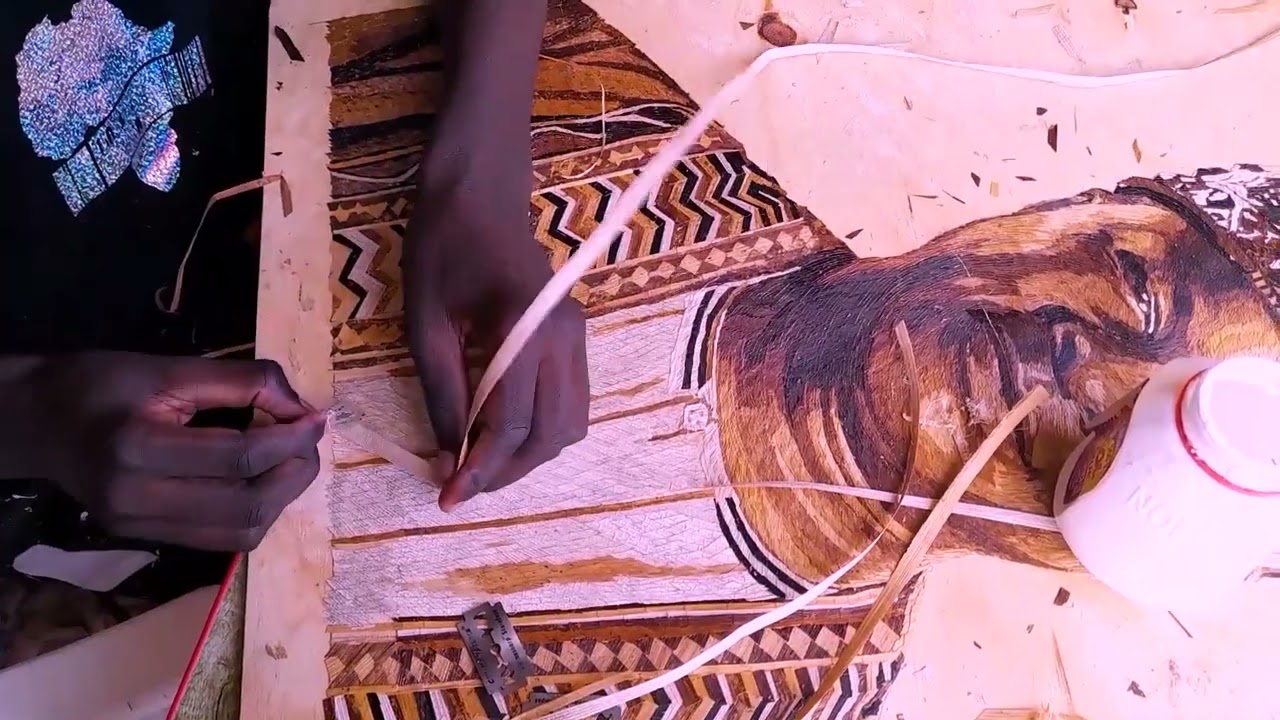The image captures a person, partially visible in the upper left-hand corner, appearing to work meticulously on a piece of artwork bordered by wood. The individual, dressed in a black shirt adorned with a blue and white emblem of Africa, is utilizing both hands in their craft. Their right hand is visible from below the shirt, while their left hand, extending from the top of the image, holds a ribbon or strip of fabric that intertwines with the artwork. This work seems to involve wood carving or shaving, indicated by the presence of a razor blade and wood splinters.

The artwork itself portrays a man with dark skin, adorned in a richly designed brown sweater and a thick-banded hat. His image tilts slightly to the right, making his head positioned on the right side and upper body on the left. The detailed sweater features various designs, and he dons a white shirt underneath. The hat is partially cut off at the top of the image and is accentuated with a red band and white element over the left eye, trailing ribbons around his neck and mouth.

The person's dark-skinned hands are working delicately on this artwork, possibly enhancing or creating the piece. The surface also hints at silver glitter, which might be part of the t-shirt's design, adding an extra layer of complexity and texture to the depiction. The individual's precise hand positions and the integration of materials suggest a careful process of crafting, whether it be carving, painting, or another form of art making.